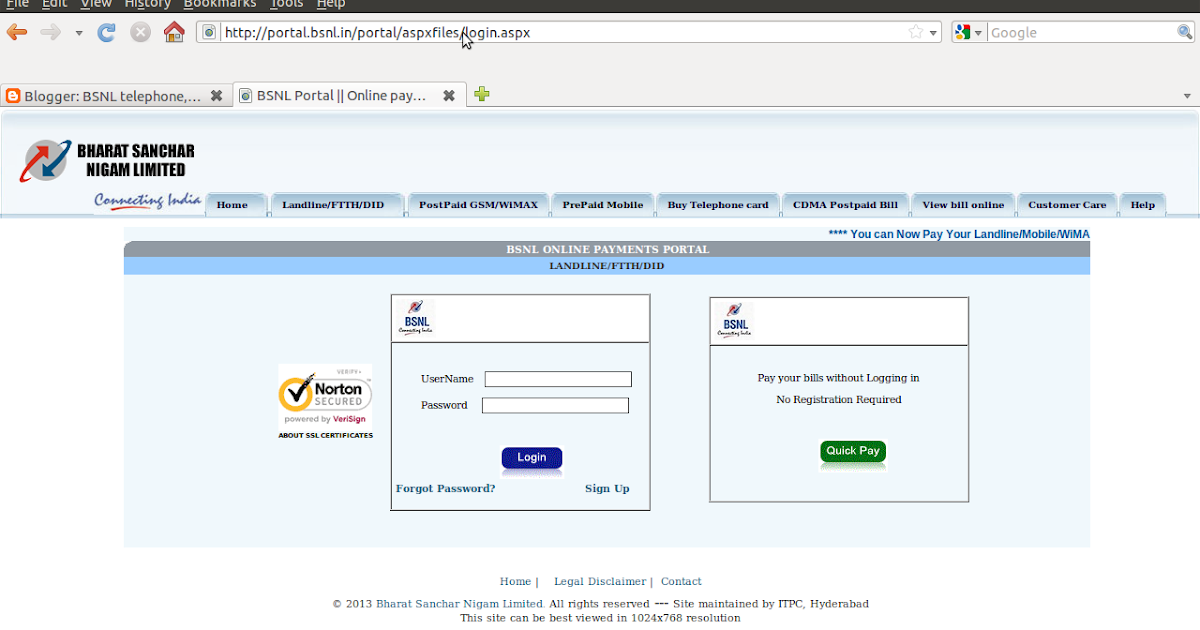This detailed caption describes an image of a payment portal page for Bharat Sanchar Nigam Limited (BSNL):

---

This image is a rectangular screenshot of a computer screen displaying a payment portal for Bharat Sanchar Nigam Limited (BSNL), a major telecommunications company in Hyderabad, India. The screenshot features a user interface with a predominantly white background, seamlessly blending with the browser window. 

At the top, there's a typical browser header in black, featuring options like File, Edit, View, History, Bookmarks, Tools, and Help. The browser's address bar displays the URL: `http://portal.bsnl.in`, followed by various suffixes.

Below the address bar, a set of navigational tabs is present. Further down, the main content area is divided into sections with a gray and blue horizontal banner. The gray banner reads "BSNL Online Payments Portal," and the blue banner reads "Landline FTTHD Ideas." Both banners are accompanied by a "Norton Secured" logo, indicating a secure connection.

The page is divided into two main boxes. The box on the left prompts users to enter a username and password for logging in. The box on the right offers an alternative method to pay bills without logging in, titled "Pay Your Bills Without Logging In: No Registration Required - Quick Pay." 

This payment portal allows users in Hyderabad to conveniently settle their bills for various BSNL services, reflecting the company's effort to streamline online payments.